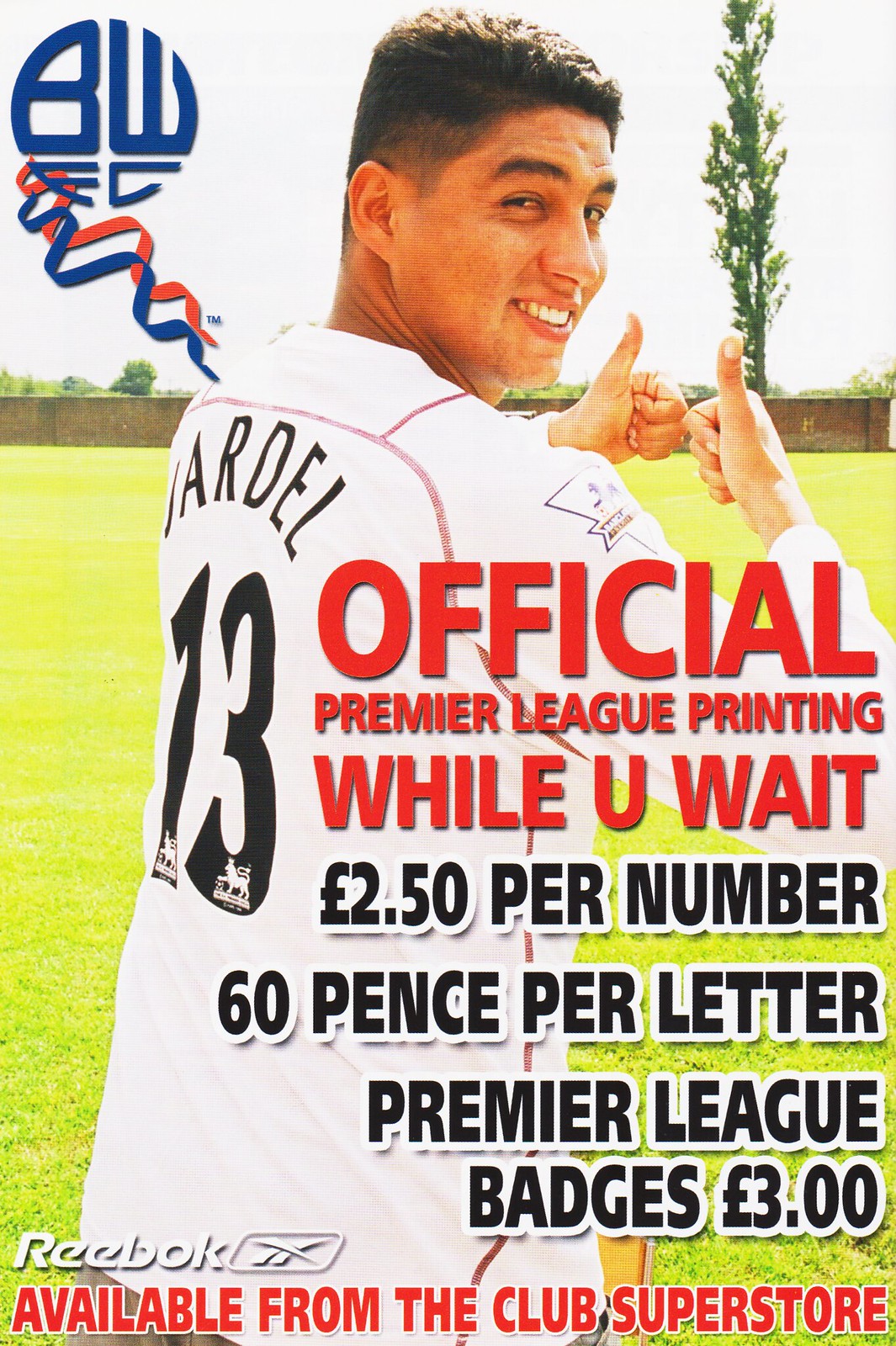A white soccer jersey-clad player, identified as Jardell from the black number 13 on his back, is captured in a dynamic pose. He stands on a green soccer field, with grass beneath his feet and a stone or brick wall and tall, thin trees in the background. The player, possibly of Indian descent, has short hair and is smiling while looking over his shoulder at the camera, giving two thumbs up. Engraved on the top left corner of the image is the logo 'BWFC,' likely representing his football club. To the right side of the image, there's marketing text in red that reads, "Official Premier League Printing While You Wait." Below that, in black, it specifies the costs: "£2.50 per number, 60 pence per letter, Premier League Badges £3." The bottom of the image features the Reebok logo along with the text 'Reebok' in white, and in red, it says, "Available from the Club Superstore."